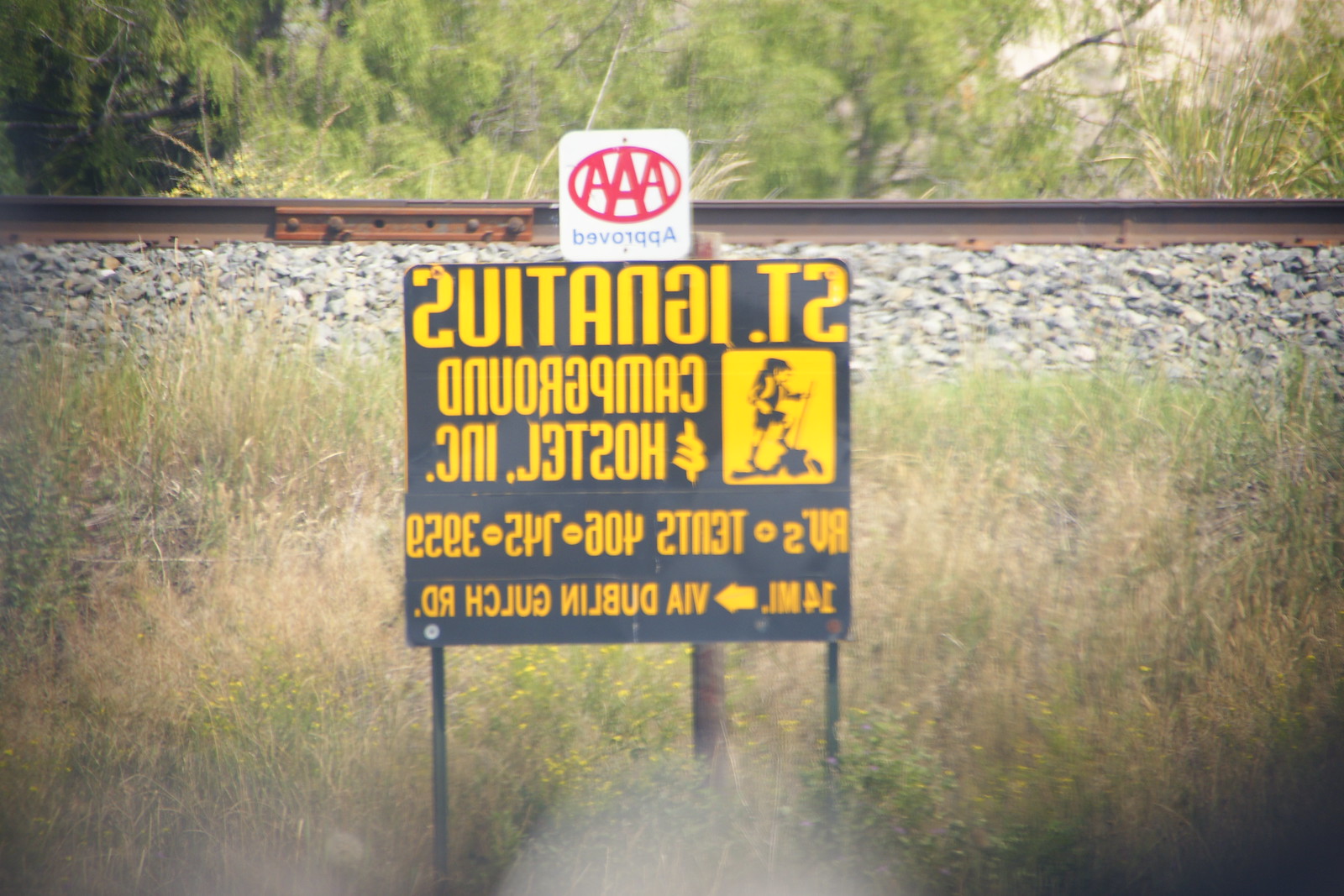The image is a slightly blurred outdoor photograph featuring a sign positioned near railroad tracks, taken from a frontal perspective. The primary sign is brown with yellow lettering and is mounted on a metal pole. The text on the sign reads "St. Ignatius Campground and Hostel, Inc." Beneath this text is a small graphic of a person hiking while holding a walking stick. Above this, there is a white square sign with a red AAA emblem that indicates "Approved." Additionally, an auxiliary sign below the main text reads "14 miles" with an arrow pointing to the right. In the distance, one can see a horizontal line of railroad tracks, flanked by a gravel bed and surrounded by medium-high grass, stretching towards the horizon.